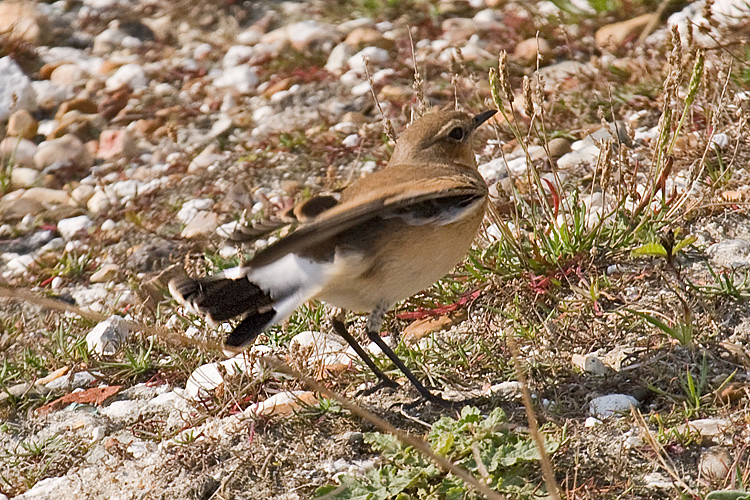This outdoor photograph captures a small, delicate bird standing on a rocky landscape interspersed with patches of grass and weeds. The foreground is blurred by two long stems of grass, directing focus to the bird. The bird has predominantly light brown feathers with darker brown around its black eyes. Under its slightly lifted wings, faint streaks of white and black are visible. Its small, triangular black beak and thin, black legs add to its fragile appearance. The tail feathers are particularly detailed, showcasing white bases transitioning to black tips. The rocky ground beneath the bird consists of stones in varying shades of white, tan, grey, and green hues from scattered vegetation, creating a rich, natural backdrop. The bird’s beak and gaze are oriented towards the upper right, adding a dynamic element to the scene.